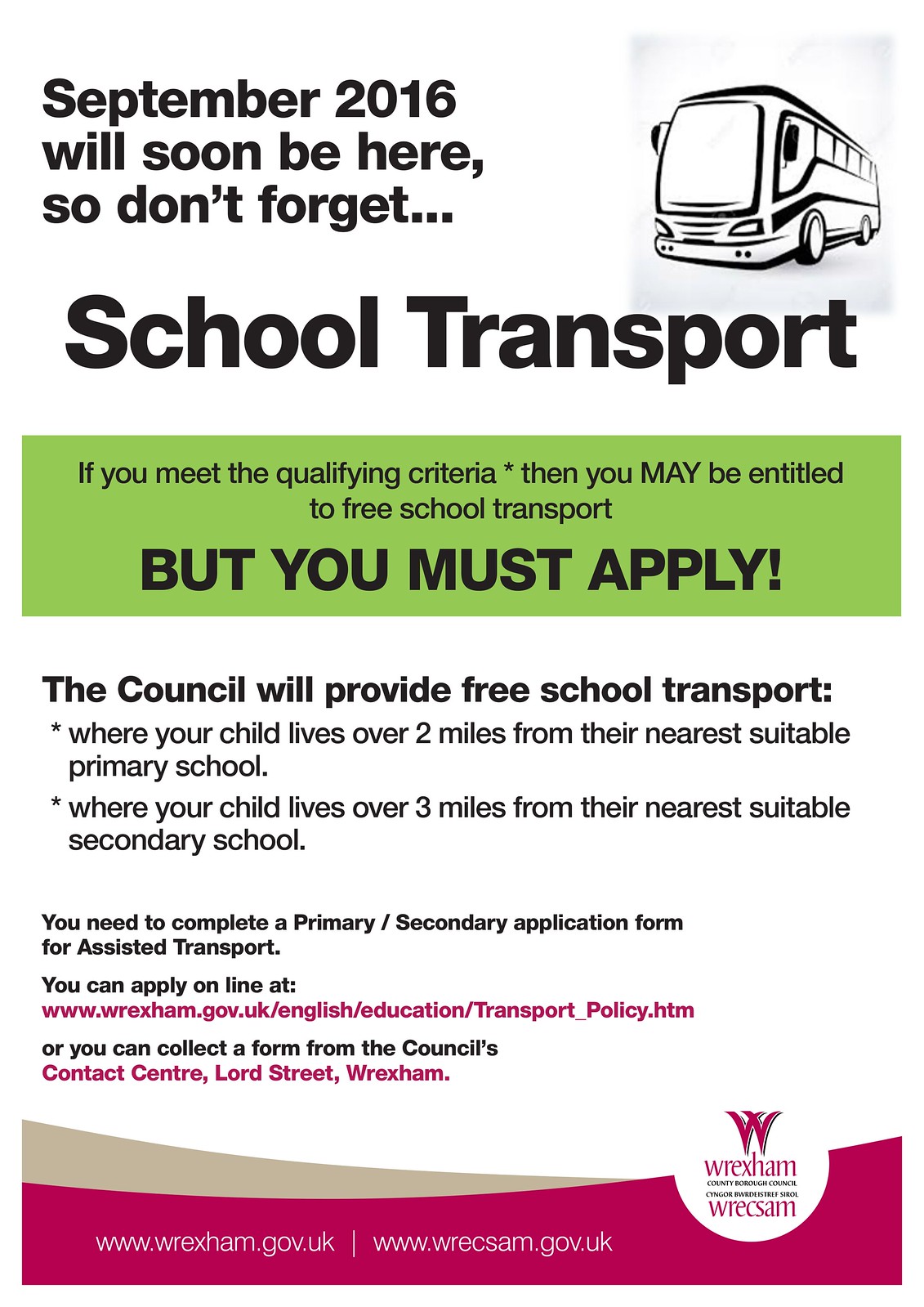The image is a notice about school transport for September 2016. The background is primarily white with various text sections in black and some highlights in green and red. At the top, in black lettering, it states, "September 2016 will soon be here, so don't forget," with a clip art image of a black and white school bus icon next to it. Underneath, "School Transport" is prominently displayed. 

Below that, within a green rectangular background and in bold black letters, the notice explains, "If you meet the qualifying criteria, you may be entitled to free school transport, but you must apply!" 

Continuing on a white background, the notice further details in black lettering that the council will provide free school transport if a child's home is more than two miles from the nearest suitable primary school or more than three miles from the nearest suitable secondary school. 

Applicants must complete a primary-secondary application form for assisted transport. The notice indicates that applications can be submitted online at a given URL (www.wrexham.gov.uk/english/education/transport_policy.htm) in red lettering. Alternatively, forms can be collected from the council's contact center located at Lord Street, Wrexham, also highlighted in red.

The bottom part of the notice features a graphic section with a white and beige curved design overlaid by a red sloping line. Within this red section, still in white lettering, the web address www.wrexham.gov.uk is repeated alongside the Wrexham Council logo.